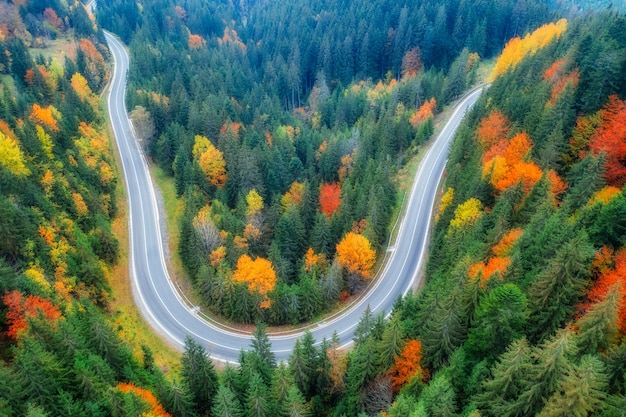This aerial photograph captures a well-maintained highway winding through a vibrant forest, creating a distinct U-shape in the center of the image. The road, devoid of any vehicles, snakes its way from the right-hand side, curves around the bottom, and continues its path up through the top. The forest is a mosaic of autumn colors with trees showcasing a range of hues from dark greens to bright yellows, oranges, and reds, giving the scene a watercolor-like quality. The point of view suggests the photo was taken from a high vantage point, possibly a helicopter, highlighting the contrast between the colorful deciduous trees near the road and the darker green coniferous trees that dominate the scene further back. The grass beneath the trees can also be glimpsed, adding another layer of complexity to this serene, midday landscape.